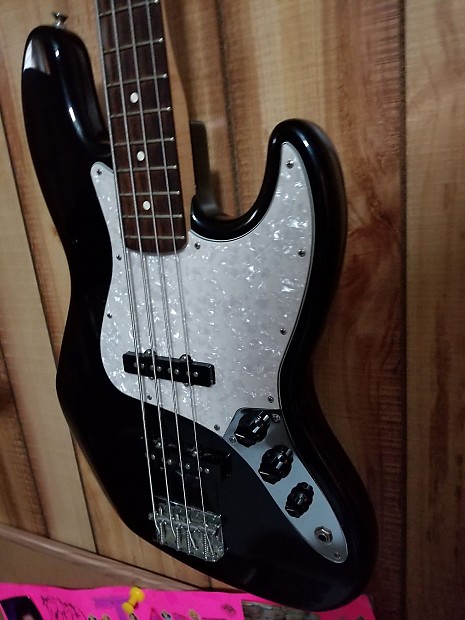This image captures an electric guitar mounted on a wooden wall with vertical paneling in medium and light brown shades. The wall recedes to the left, creating a sense of depth, with a brown baseboard visible along the bottom-left edge. At the very bottom, a bright pink object with black areas peeks into the frame from the left. The right-hand fourth of the image is filled with uninterrupted wooden paneling. The guitar itself hangs prominently, only partially visible, featuring a shiny black finish and a striking marbled white area on the right side, extending towards the lower right. The guitar's shape is curvy and reminiscent of an hourglass, with the marbled white area outlined by the surrounding black.